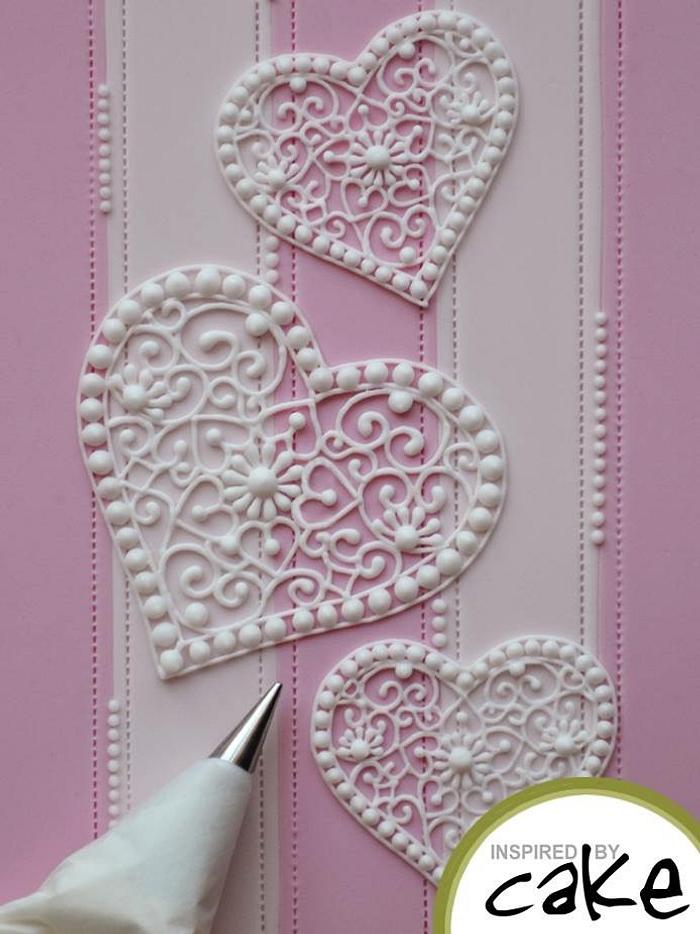The image depicts a detailed and intricate cake decoration design featuring three white hearts on a pink and white vertically striped background. Each heart is uniquely adorned with abstract patterns and latticework, bordered by circles or beads that appear to be made from icing. There are nine to ten tiny white dots along the borders where the pink and white stripes intersect, mimicking the appearance of stitches. The hearts are arranged artistically, with the largest heart in the center slightly leaning to the right, a medium-sized heart at the top angled to the left, and another medium-sized heart at the bottom positioned vertically. In the bottom right corner, a semicircle with several shades of green encircles the phrase "INSPIRED BY CAKE"—the words "inspired by" are in gray and capitalized, while "cake" is in a black, handwritten-style font. Additionally, on the bottom left, there is a white cake piping pen with a metal tip, indicating the use of a cake decorating kit for creating these designs.